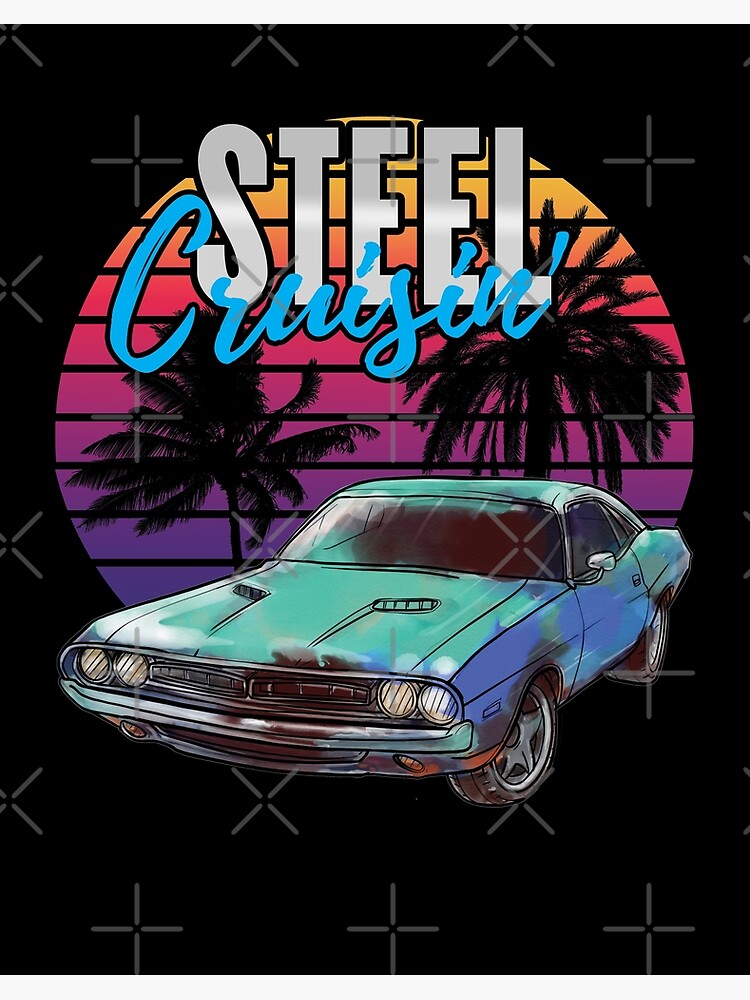This stylized poster, reminiscent of 1980s retro designs, features the bold caption "Steel Cruisin'," with "Steel" in large, bold white letters and "Cruisin'" in a light cyan blue script. The focal point of the poster is a classic vintage muscle car, seemingly a Dodge Charger, in a striking teal color with a green top and blue sides. The car is fully intact, with no damage or rust, and sports chrome bumpers and white-walled tires. Behind the car is a circular image with two black and white palm trees, set against a vibrant gradient sky that transitions through purples, blues, oranges, and yellows. The background of the poster is black, adorned with an array of small white crosses, X's, and plus signs, creating a dynamic and textured visual effect. The poster's design is evocative of a blend between contemporary and retro styles, capturing a nostalgic yet modern vibe.